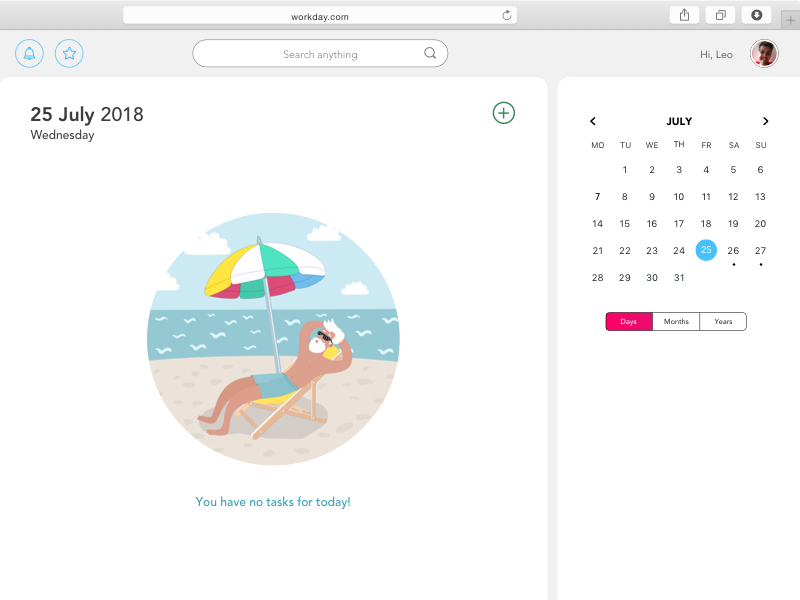This screen capture from workday.com prominently features an organized and user-friendly interface. At the top, a thin gray stripe spans horizontally, immediately below which lies a white search box accompanied by a small gray arrow. Adjacent to this search box, within the same thin gray stripe area, are three white squares each containing distinct icons: the first depicts a square with an up arrow, the second a stack of paper, and the third a black circle with a downward-pointing white arrow.

Descending further on the interface, a pale gray box is noticeable on one side. Here, two circular blue icons stand out – one featuring a bell and the other a star. Adjacent to these is the white search box repeating from above. To the right is a personalized greeting, "Hi Leo," accompanied by a smiling profile picture. Below this greeting, in bold black text, the date "25th July 2018, Wednesday" is indicated, accompanied by a whimsical illustration – a cartoonish white-haired, white-bearded man with black sunglasses lounging in a yellow beach chair on a white sandy beach. The scene is complete with a vibrant umbrella composed of yellow, white, green, red, and blue segments. The man, dressed in blue swim trunks, relaxes beside blue-gray waters with white-capped waves, beneath a serene blue sky dotted with fluffy white clouds. Additionally, a blue plus sign within a circle is visible to the side of this image, under which the text in blue reads, "You have no tasks for today."

On the opposite side of the screen, a black calendar for July is displayed, highlighting July 25th with a blue circle. Below the calendar, three tabs labeled "Days," "Months," and "Years" are presented, with the "Days" tab emphasized in pink.